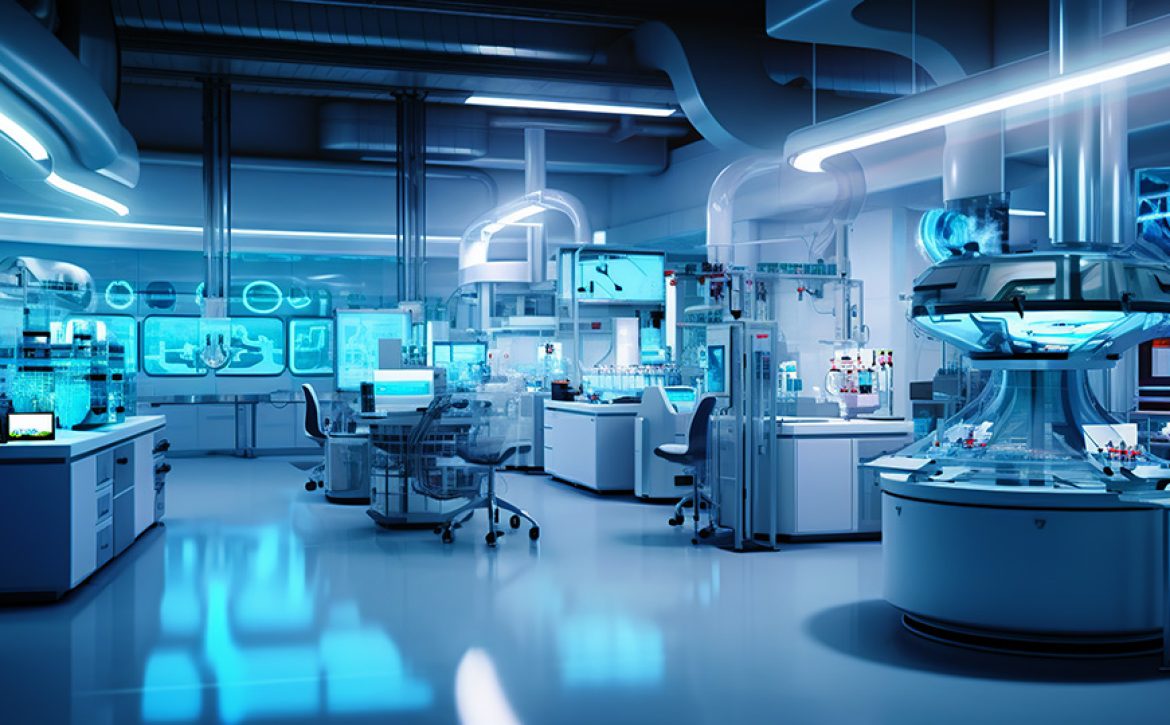The image depicts a highly futuristic and meticulously clean lab, characterized by its bluish, silver, and chrome color scheme. The floor is a bright, polished silver or gray, reflecting the ample blue lighting throughout the space. The lab features a cluttered arrangement of scientific equipment, including various devices, monitors with blue screens displaying data, and high-tech medical or experimental apparatus. Stations consist of counters and tables, each accompanied by wheeled and flat chairs. Tubular and square heating and ventilation vents are visible across the ceiling. Despite the pristine and high-tech appearance, the photograph reveals no people, leaving the function of many objects indiscernible due to the far-back angle of the shot, immersing viewers in a scene that could easily belong to a sci-fi movie or TV show.